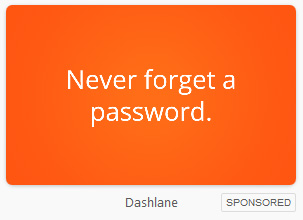The image appears to be a digital screenshot, possibly taken from a computer or mobile device screen. Dominating the top portion of the screenshot is a bright orange rectangular area with slightly rounded edges. Centrally located within this orange section are two lines of text: the first line reading "Never Forget A" and the second line reading "Password." Below this prominent orange area is a smaller gray section that extends slightly upwards to frame the left, right, and very top edges of the rectangle.

Within the middle of the gray section at the bottom, there is text in light gray reading "Dash Lane." Below this, in the far right corner, is a click-worthy rectangular button outlined in gray, with the word "Sponsored" written in gray text within it. The design is minimalist, with no additional images or text beyond the lower gray banner. The overall composition is clean and straightforward, focusing mainly on the orange rectangle with an informative message.